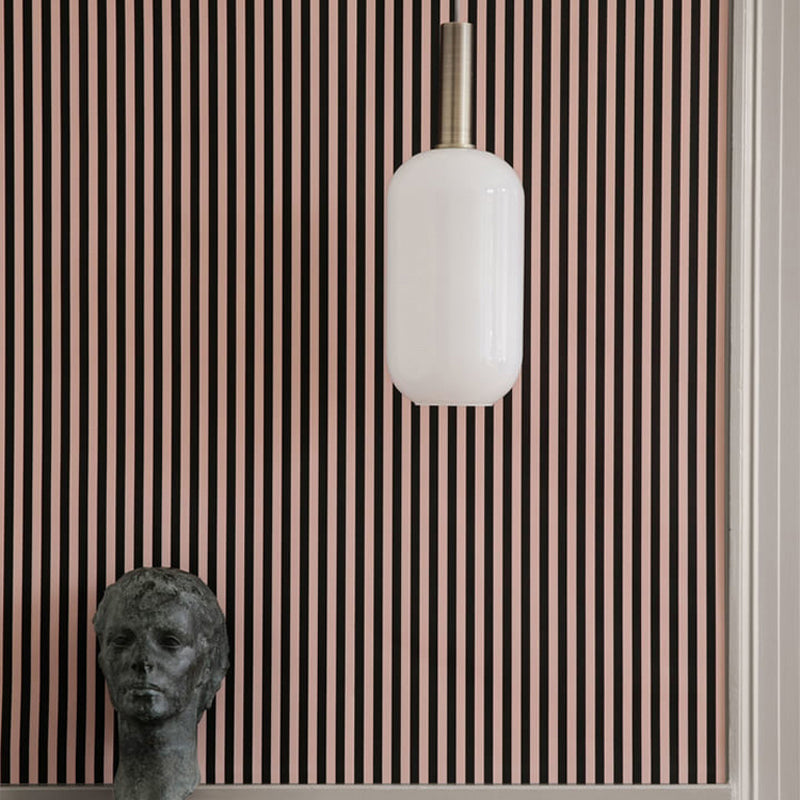The photograph captures a detailed and layered scene with distinct elements. The background wall is dominated by a surface featuring a dense pattern of tightly spaced, thin vertical tan lines with black spaces in between, evoking a striped effect. A narrow strip along the bottom and the right edge of the frame is bordered with white wooden molding. Positioned in the lower left-hand part of the image, in front of this striped background, is a small, realistic stone head sculpture of an androgynous human face with short hair. The sculpture's dark material, possibly bronze or iron, stands out against the lighter backdrop. From the top edge of the photograph, a long, narrow cylindrical black brass light fixture descends, suspending a large white glass cylinder with rounded ends—a light that has a milky, cloudy appearance. The combined elements of sculptural art, intricate background, and unique lighting create a balanced and visually compelling composition.